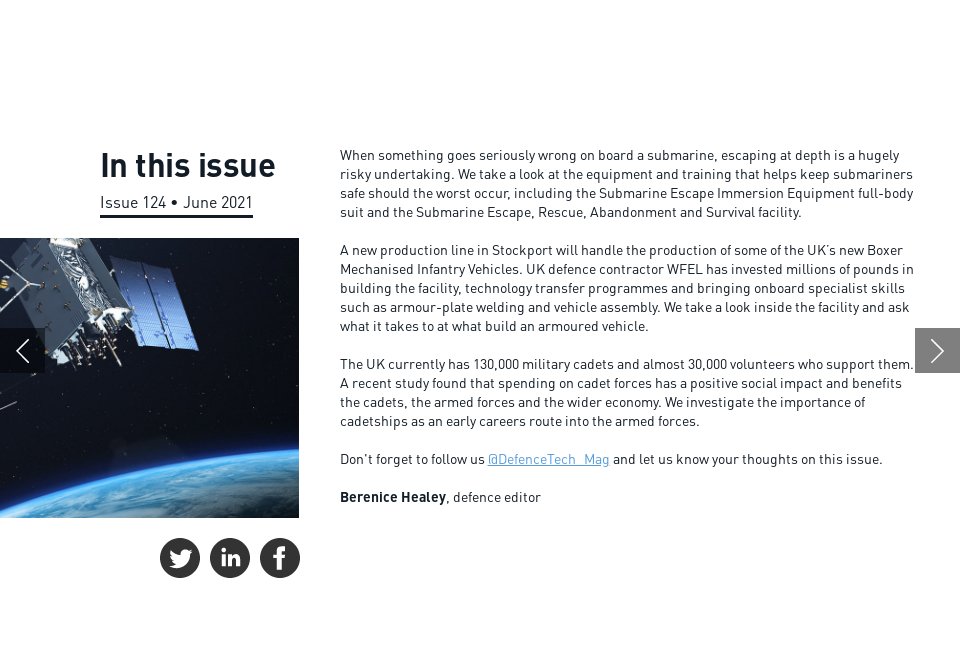This screen grab from Defense Tech Magazine showcases a detailed cover page with a minimalist design. Predominantly featuring a white background with black lettering, the layout incorporates a photograph on the left-hand side, depicting a satellite hovering above Earth. The satellite, square in shape, is oriented downwards.

On the left third of the screen, the text reads: "In this issue," followed by "Issue 124, June 2021." Below this, social media icons for X (Twitter), LinkedIn, and Facebook are displayed.

The cover also includes an introductory paragraph discussing the challenges of submarine escapes at depth. It highlights the equipment and training designed to ensure the safety of submariners in dire situations, mentioning the Submarine Escape Immersion Equipment, a full-body suit, and the Submarine Escape Rescue, Abandonment, and Survival Facility.

The next section details a new production line in Stockport dedicated to manufacturing the UK's new Boxer mechanized infantry vehicles. UK defense contractor WFEL has invested millions in constructing this facility, transferring technology, and onboarding specialized skills such as armor plate welding and vehicle assembly. Insight into the facility's operations and the process of building an armored vehicle is provided.

Another paragraph focuses on the UK's 130,000 military cadets and nearly 30,000 volunteers who support them. A study revealing the positive social impact and benefits of cadet forces for cadets, the armed forces, and the broader economy is discussed. The importance of cadetships as an early career path into the armed forces is explored.

Finally, readers are prompted to follow Defense Tech Magazine on social media and share their thoughts on the issue. The caption is signed off by Bernice Healy, Defense Editor.